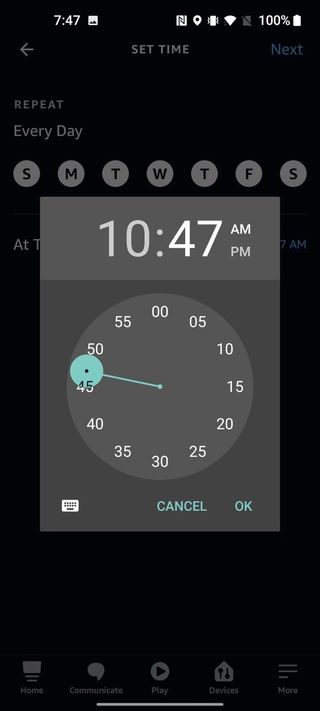The image displays a smartphone screen in dark mode, characterized by a predominantly black background. At the top left corner, the time is shown as 7:47, while the top right corner indicates a fully charged battery at 100%, alongside various other status icons. Below this status bar, the screen features the text "Set time" in light gray, flanked by a back arrow on the left and the word "Next" on the right.

Further down, the screen presents the word "Repeat" on the left, underlined by "Every day" in gray text. Beneath this, there is a row of seven circles, each marked with the first letter of the respective day of the week: S, M, T, W, T, F, S.

The central part of the screen showcases a gray box with a circular time selector. At the top of this box, the time is displayed as 10:47, with "AM" prominently highlighted. The time selector is designed with increment marks for every five minutes, ranging from 00 to 55, encircling the dial. A light blue line extends from the center of the clock to a light blue circle positioned at the 47-minute mark. At the bottom of the gray box, there are two buttons offering the options to "Cancel" or "OK."